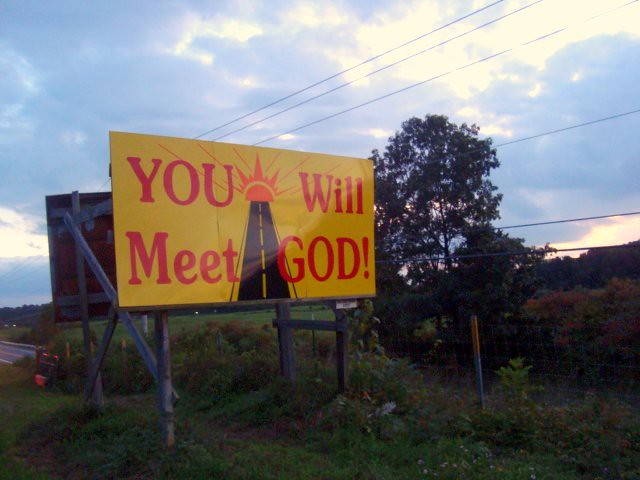The photograph captures a yellow billboard with bold red lettering that reads, "You Will Meet God," and features an illustration of a black highway extending towards an orange sun with radiant beams. The billboard, mounted on what appear to be wooden posts, is set against a backdrop of a grassy area, dense with bushes and trees. Behind it, power lines stretch across the scene. A second billboard is visible in the distance, though only its backside is seen. The roadway in the background is mostly hidden by the greenery and rolling hills, hinting at a two-lane highway. The sky above is a mix of blue and gray, with clouds indicating a cloudy, yet sunlit day, potentially close to dusk. Additionally, a yellow-painted ground marker is noticeable to the right of the billboard, adding to the detailed setting. The overall ambiance suggests a typical Southern roadside scene, likely intended to inspire viewers with its religious message.